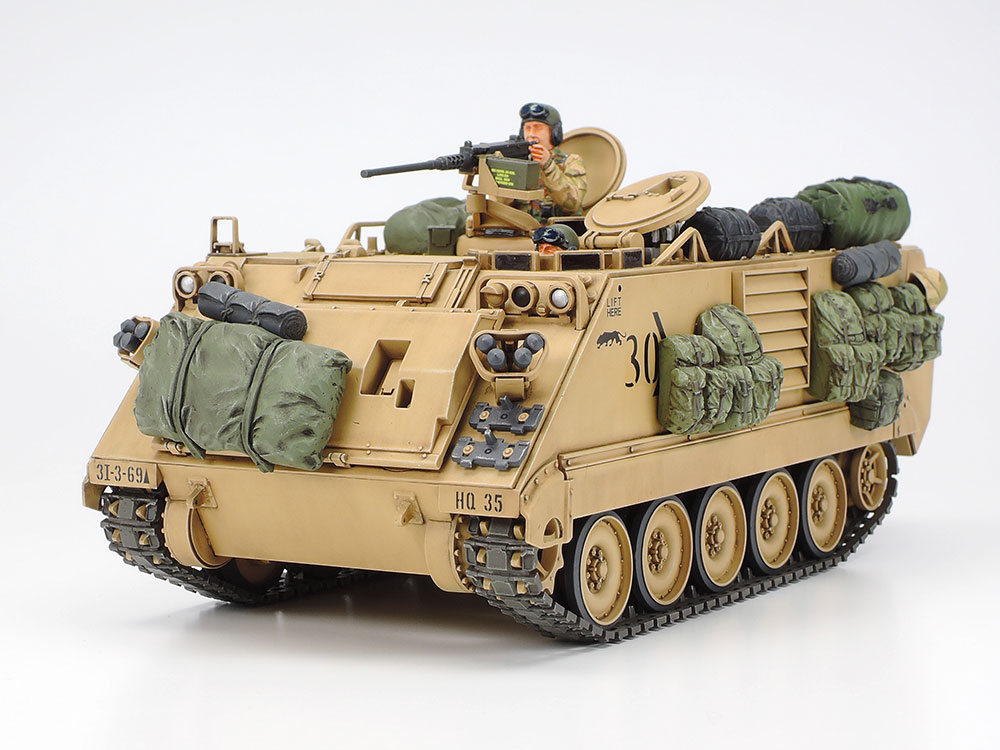In this image, we see a detailed model of a retro military tank, showcasing intricate features that hint at its status as a replica or toy. The tank, in a wheat tan color, stands prominently against a stark white table and background, emphasizing its fine details. It is equipped with large wheels, coated in wheat brown with black outer rims, all connected by metallic gray tracks that resemble those found on real military tanks. Adorning the tank are various accessories, including several dark green army bags—a mix of duffel bags and backpacks—strategically strapped to the front, sides, and top. Additionally, a rolled-up gray mat and a few black bags are visible on top of the tank.

The tank bears distinctive markings: the number "30" alongside the silhouette of what may be a tiger or panther on the side, "HQ 35" on the front, and "3T-3-69" accompanied by a triangle on another section. There is also a "Lift Here" label on the side emblazoned in black text.

A soldier figurine, reminiscent of a GI Joe, is positioned at the top of the tank. He wears a dark green helmet with goggles and brown army fatigues. The soldier holds a black machine gun, mounted on the tank and aimed as if he’s scanning for threats. In front of him sits a green ammunition box marked with yellow writing, adding to the authenticity and detail of the scene.